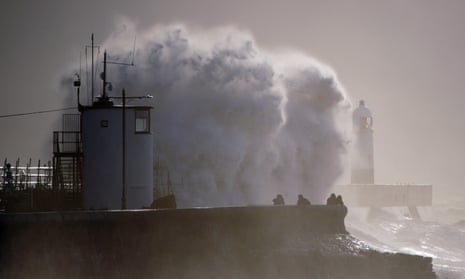The black-and-white photograph presents a dramatic and tumultuous shoreline scene dominated by an explosive plume of water smashing against a cliff or concrete wall. On the far right, ferocious waves create a chaotic blend of white and gray froth, suggesting a storm or disaster. Amid the violent sea, a small lighthouse stands at the end of a jutting dock, barely discernible through the mist and crashing water. The left side of the scene features a cylindrical structure, possibly a tower attached to a network of pipes, power lines, and antennas, all contributing to the industrial atmosphere. Shadows of onlookers are visible along the edge of a compound wall, gazing at the formidable display of nature. Overhead, the sky is uniformly gray, enhancing the monochromatic and eerie ambiance of the scene.